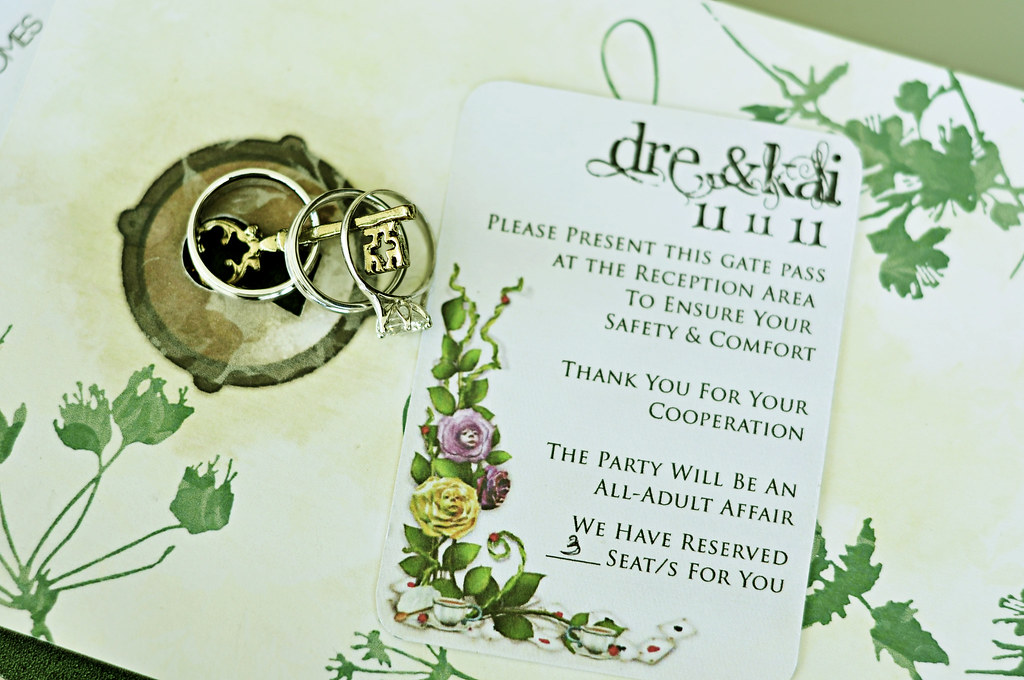The image showcases a party invitation set upon a decorative white surface adorned with green floral and ivy illustrations, concentrated primarily in the bottom and top right corners. The invitation, addressed to Dre and Kai, reads: "Please present this gate pass at the reception area to ensure your safety and comfort. Thank you for your cooperation. The party will be an all-adult affair. We have reserved three seats for you." The text "D and K" followed by "11-11-11" is prominent. Adjacent to the invitation is a stylized illustration of a circular key ring with a key threaded through three smaller circular rings, giving it an antiquated appearance. This illustration is bordered by a dark green circle. The background of the invitation also features subtle details resembling faint coffee stains, adding a touch of vintage charm to the overall presentation.